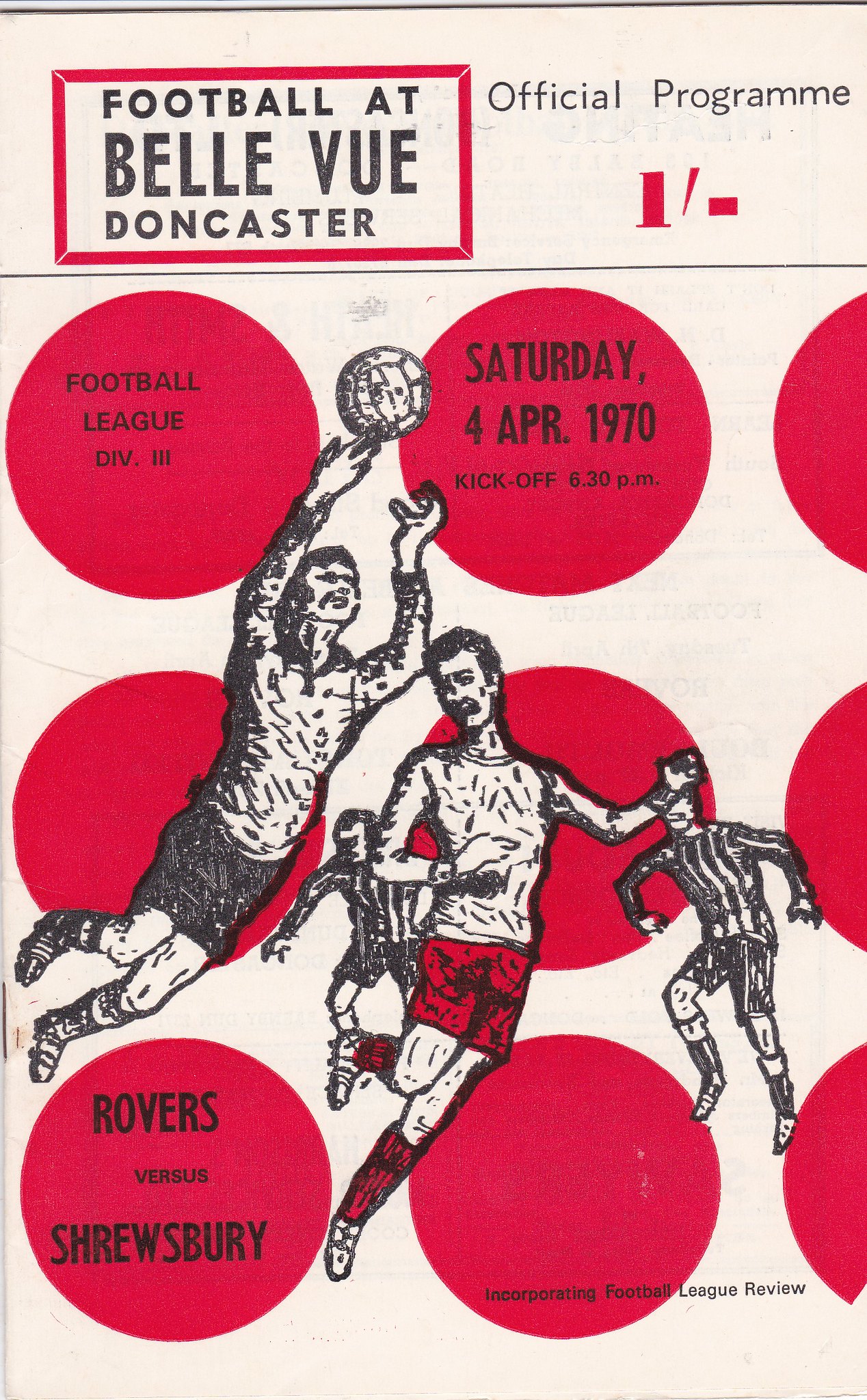The image depicts the front cover of an official program for a soccer game at Bellevue, Doncaster. The program cover is vertically rectangular with a predominantly white background adorned with several red circles, which mimic the pattern of a soccer ball. A black line runs horizontally above these circles, setting apart the title text. In the upper left corner, a red-bordered rectangle contains the text "Football at Bellevue, Doncaster", while the upper right corner features the phrase "Official Program." Positioned centrally, the cover showcases illustrations of three soccer players, one of whom is dressed in red shorts and socks, alongside a referee in a striped shirt and shorts. Additional circles on the cover provide more details: one states "Football League Division 3," another indicates "Saturday 4 April 1970, kickoff 6.30 p.m.," and a third at the lower left reads "Rovers vs. Shrewsbury." In the lower right corner, small text mentions "Incorporating Football League with You." The overall color scheme of the cover includes white, red, black, and gray, emphasizing the official and historical nature of this soccer event.